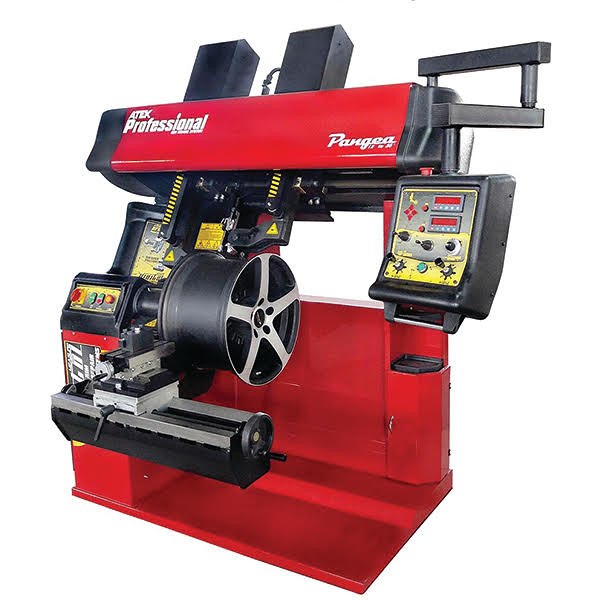Here is an image of a very advanced and unique machine, primarily red with black accents and labeled "ATEX Professional." The machine features a control panel on the right and additional controls on the left. At its center, there is an intricate hub resembling a wheel designed for an exotic car, flanked by a lathe-type setup indicative of a manufacturing process. The machine appears to be engineered for crafting high-end aluminum or alloy wheels for luxury vehicles. The cursive text "PANGEA" is also visible on the machine. This high-tech, complex device includes various switches and mechanics, underscoring its specialized and sophisticated nature.